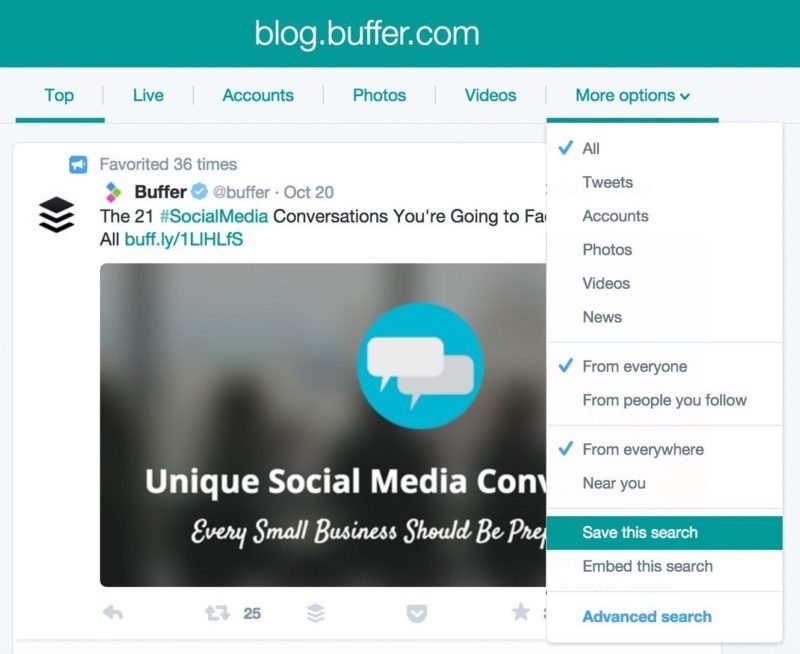This image appears to be a screenshot from a webpage, specifically of a blog post on the website blog.buffer.com. At the top of the screen, a green navigation bar displaying the website’s URL, `blog.buffer.com`, is visible.  

Below this bar, there is a horizontal menu with several clickable categories labeled, from left to right, as: Top, Live, Accounts, Photos, Videos, and More Options. The 'More Options' has been clicked, revealing a drop-down menu on the right side of the screen. This drop-down menu lists several filters and actions in the following order from top to bottom: All, Tweets, Accounts, Photos, Videos, News, From Everyone, From People You Follow, From Everywhere Near You, Save This Search (highlighted), Embed This Search, and Advanced Search. There are checkmarks next to the options 'All', 'From Everyone', and 'From Everywhere'.

The drop-down menu slightly obscures the right side of the page, but on the left side, a tweet can be seen. This tweet has been favorited 36 times by Buffer on October 20th. The visible portion of the tweet reads: "The 21 social media conversations you’re going to…", and it is partially covered by the drop-down menu. 

Beneath the tweet's text is a link, `allbuff.ly/1lihlfs`. Below that, there is an image consisting of two text bubbles inside a circle. The visible text within this image reads: "Unique social media con...", and "every small business should be pre...". The full text is not visible due to the drop-down menu covering part of the image.